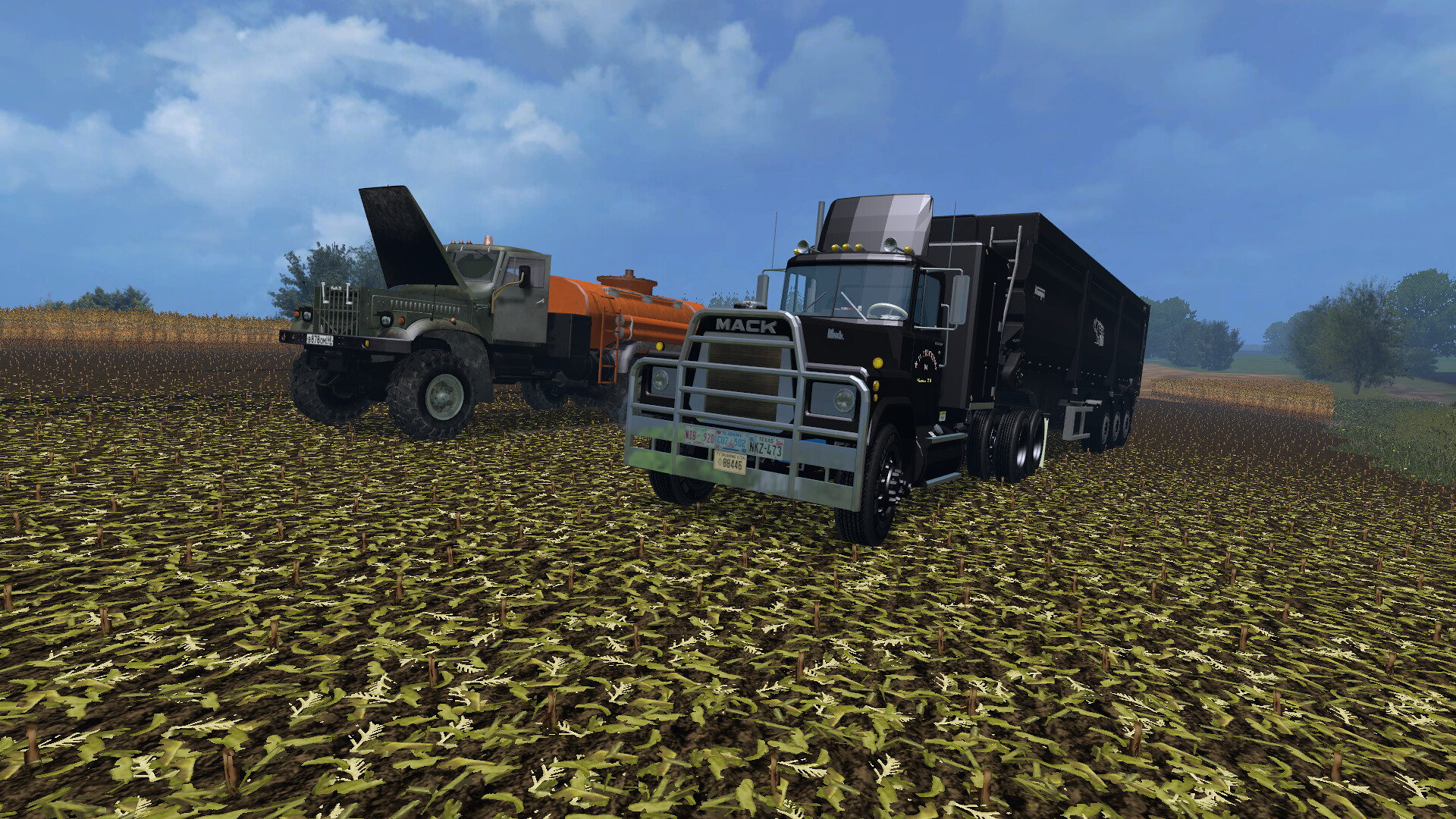The image is a horizontal rectangular computer-generated animation depicting a farming scene. In the center are two prominent trucks positioned diagonally, resting on a textured green field dotted with small white flowers. The crop, which appears to have been recently cut down, possibly corn or soybeans, still maintains a dark green hue. The sky above is vivid blue with scattered white clouds. 

The truck on the left is a tanker truck featuring a silver cab with its hood raised, and an orange liquid tank at the back. The one on the right is a freight truck with a black-painted cab and trailer, and a silver grille on the front. The truck bears the name "MACK" in silver letters on the hood and has a white license plate. The background reveals another field with yellow stalks likely indicating a different crop, and beyond that, a line of trees. On the left side of the image, an additional field and more trees frame the scene. The detailed textures and realistic rendering reinforce the image’s computer-generated nature.